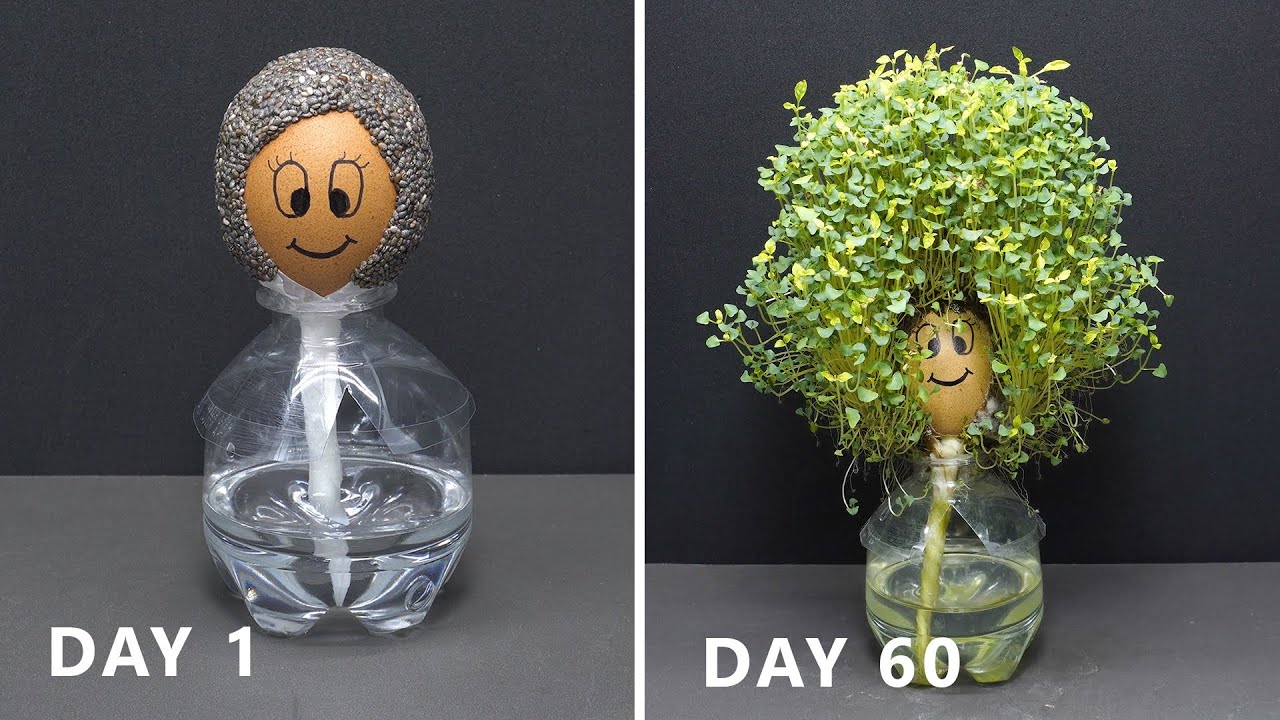The image features a side-by-side comparison of a Chia Pet's growth over 60 days. On the left, labeled "Day 1," there's a small, exaggeratedly smiling Chia Pet with large eyes, housed in a clear plastic bottle half-filled with water. The bottle has been horizontally cut, and a straw extends into the water, supporting the Chia Pet, which looks like a brown egg coated with dark gray and black seeds poised to sprout into hair. The background is dual-shaded, with a dark gray upper half and a lighter gray lower half. On the right, labeled "Day 60," the same Chia Pet is shown, now crowned with a dense, lush growth of green and yellow sprouts, its smile still beaming. The water has turned a yellowish-green, slightly less full than before, but the transformation is striking. This detailed visual showcases the impressive progress, symbolizing either an advertisement or a proud display of personal Chia Pet cultivation.